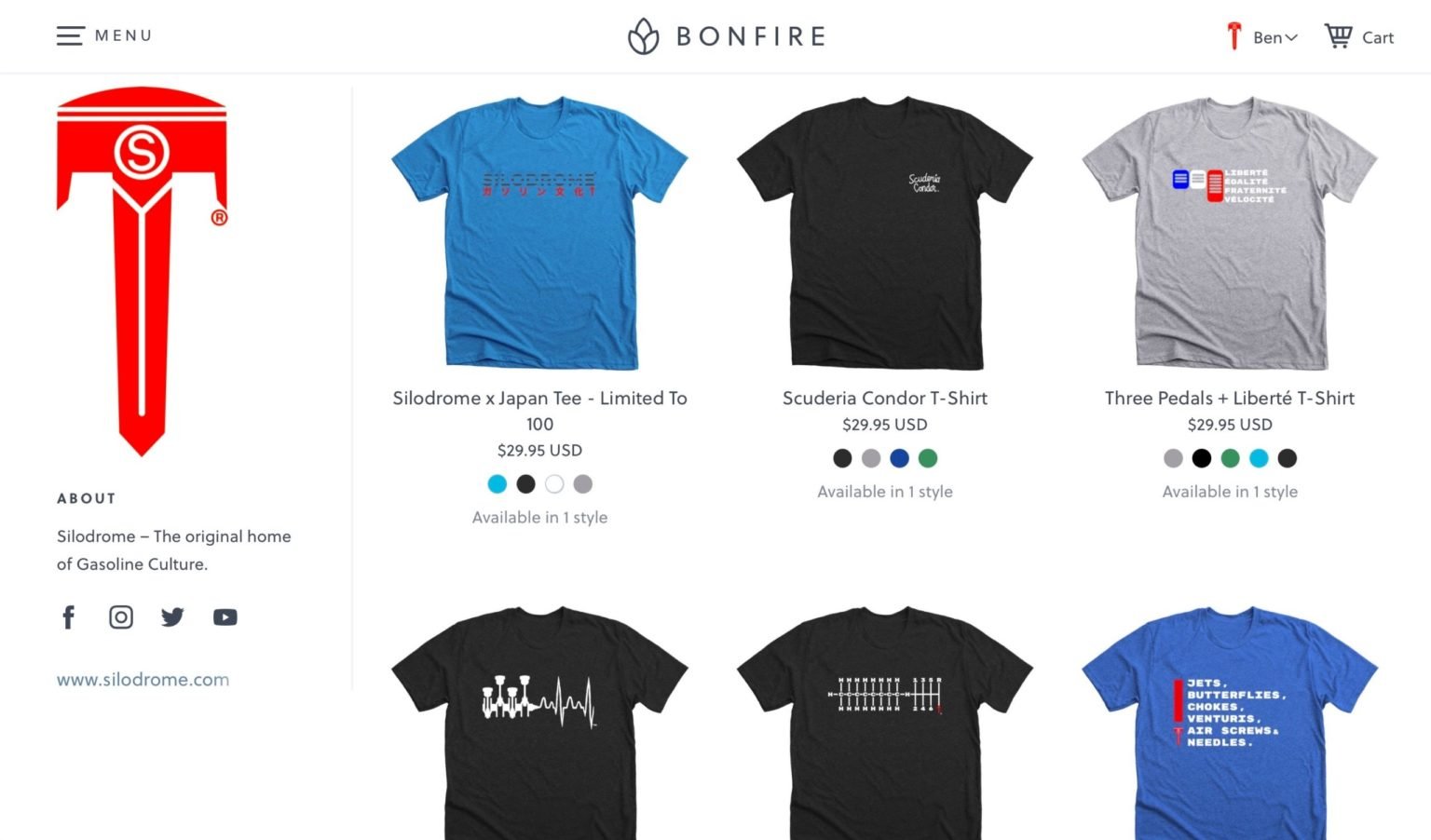This image showcases a webpage with a clean, white background. At the top left corner, the word "Menu" is displayed. Centrally aligned at the top is an elegant black illustration of a plant, accompanied by the text "Bonfire." Towards the top right, the name "Ben" is visible with a downward arrow beside it, and further to the right is a shopping cart icon labeled "Cart."

Beneath this header section, six different t-shirts are featured. The top left shirt is blue with unidentifiable text on its front, too small to be clearly read. Another notable shirt is labeled "Silodrome X Japan T - Limited to 100," priced at $29.95 USD. This shirt is available in four colors: blue, black, white, and gray, and it is indicated to be available in one style.